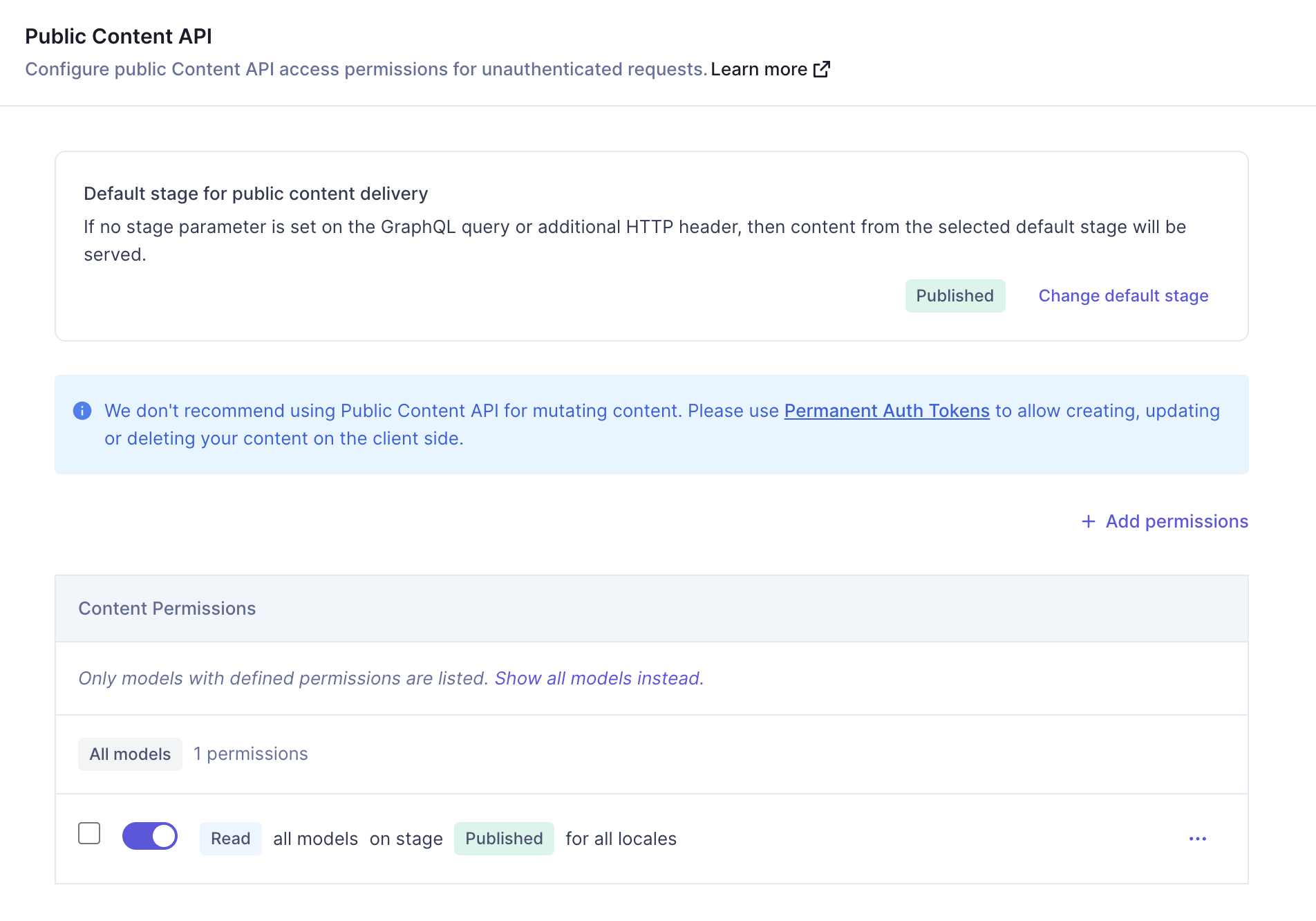In the image, a web interface is displayed against a white background. At the top, there is a header that reads "Public Content API." Below this header, a description states, "Configure public content API access permissions for unauthorized requests."

Centering the screen is a blue square containing a smaller blue circle. Below it, a subheader indicates, "Default stage for public content delivery." An explanation follows: "If no stage parameter is set on the GraphQL query or additional HTTP header, then content from the selected default stage will be served." A "Learn more" link with an icon featuring an up arrow is provided for further information.

To the right, a prominent blue "Publish" button is visible, accompanied by a "Change Default Stage" button. Another button with an up arrow and three horizontal lines features the label "Sort by model A to Z." A "Plus Filter Permissions" button appears below, alongside a blue button labeled "Plus Create Permission."

Further down, a blue box titled "Content API Permissions" includes a down arrow at its end, indicating a collapsible section. The text within states, "Only models with defined permissions are listed. Show all models instead."

At the bottom of the interface, there is a box labeled "All Models: 1 Permission." This box contains a small blue toggle button, a "Read" label, and a statement that reads, "All models on all stages with all locales." Finally, three vertical dots signify additional actions or settings.

The comprehensive layout ensures users can manage and configure permissions for public content effectively and intuitively.